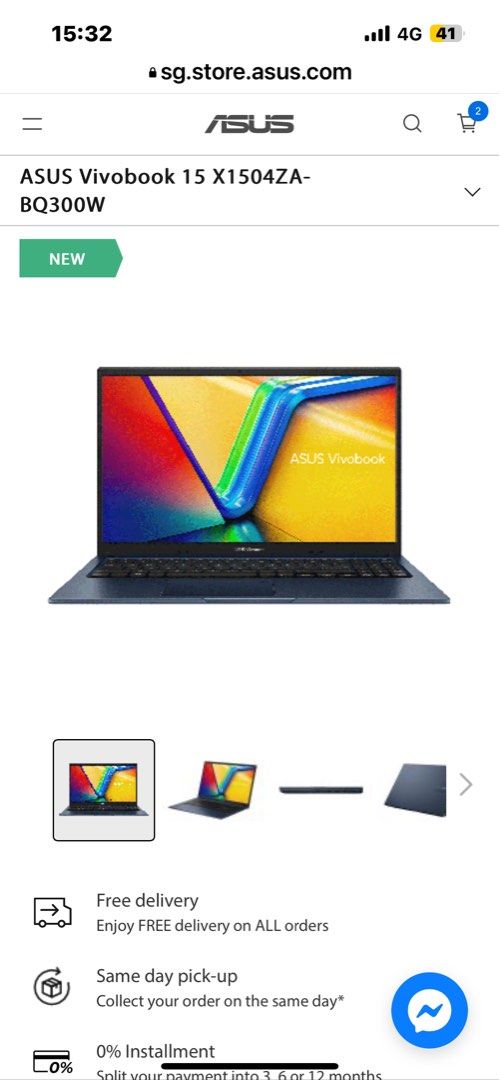The image depicts a screenshot of the sg.store.asus.com website viewed on a mobile device. At the top of the screen, the time is displayed as 15:32, alongside a 4G signal indicator and a battery level icon showing 41% charge. In the top right corner, there is a shopping cart icon and a magnifying glass icon, signifying the options for viewing the shopping cart and searching the site, respectively. Centered prominently is the ASUS logo.

Beneath this header, the page features an ASUS Vivobook 15 laptop. The laptop's screen displays a vibrant wallpaper with an abstract pattern composed of intersecting lines in various colors, including red, blue, yellow, green, dark blue, and orange. To the right of the laptop is a green rectangular box with the word "NEW" labeled on it, indicating the product's release status.

Below the main image of the laptop, there are additional images showcasing different angles of the device, offering a comprehensive view of its design. Furthermore, there are three icons beneath these images: a truck symbol indicating delivery options, a "Same Day Pickup" icon, and a "0% Installment" icon, presumably highlighting payment options available for the product.